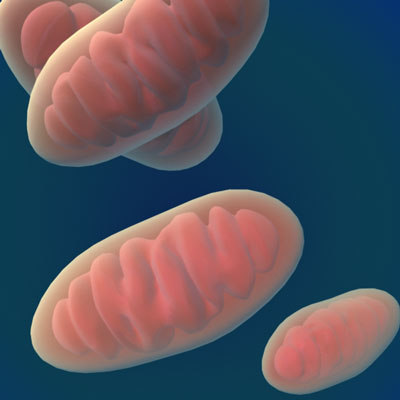The image features a computer-generated depiction of four translucent, beige, oval-shaped cells, resembling footballs or loaves of bread. These cells are set against a dark blue background, with their interiors filled with a pink, intestine-like substance. The composition appears disorganized, as the cells are scattered across the image without a central focus. This detailed and vivid portrayal is reminiscent of what one might observe under a microscope in a scientific, medical, or educational setting, such as a hospital, medical school, or chemistry lab. This image could potentially be used in a PowerPoint presentation or as part of an educational slide to illustrate biological materials or cellular structures.